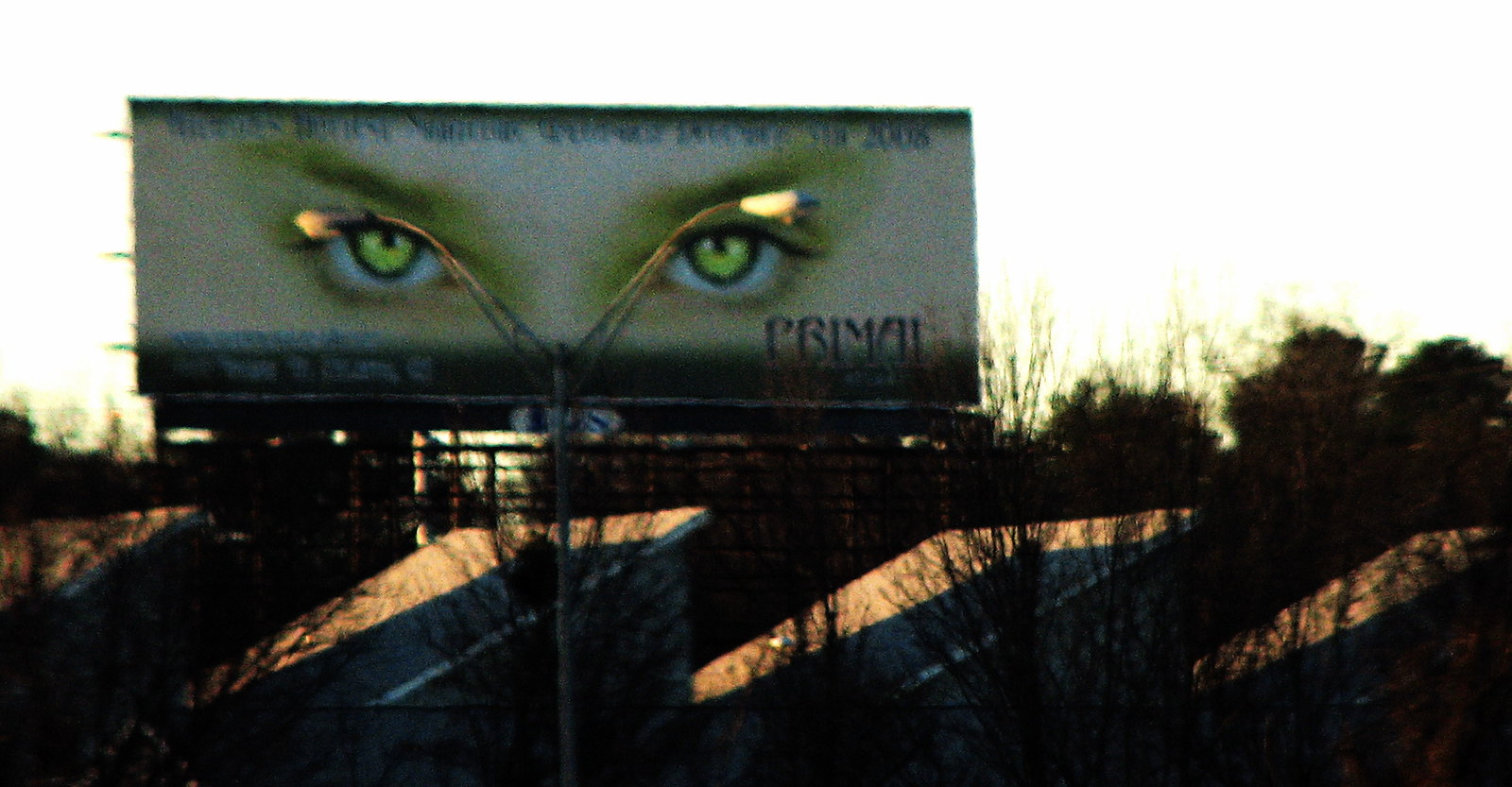This image features a billboard set against a backdrop of rooftops and leafless trees. The billboard stands out with its light gray background and a striking depiction of light lime-green eyes, complete with dark blue pupils. Around the irises, there is a distinct ring of darker blue. Above the eyes, green eyeshadow extends elegantly over the eyebrows. Blue text is present at the top of the billboard, though it is too small to decipher. The word "Primal" is conspicuously positioned in the right-hand corner. A streetlight in front of the billboard appears to illuminate the eyes, creating an impression that the lights are integrated into the display itself. Behind the billboard, rooftops on a steep slope, likely belonging to houses or other buildings, add depth to the scene. The trees in the background are bare, devoid of any leaves.